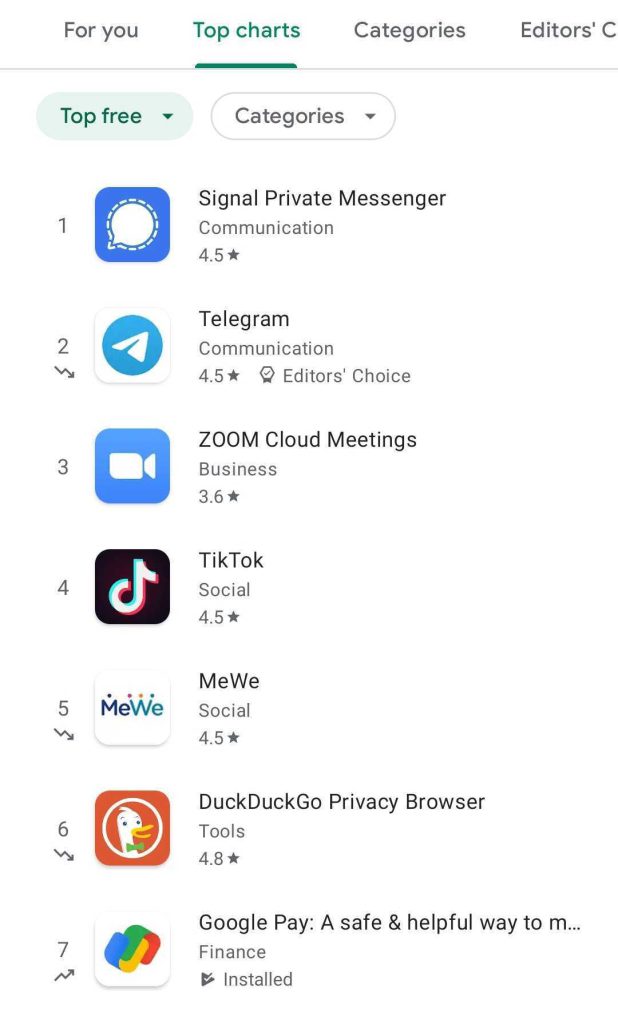This image is a portrait-mode screenshot with a predominantly white background. At the top left corner, there are several menu options including "Top Charts," "Categories," and "Editors' Choice," although "Editors' Choice" is partially cut off and might require scrolling to the right to view fully. The "Top Charts" option is currently selected, evident by its green underline and highlighting.

Below the menu, there are two buttons side-by-side. The left button, labeled "Top Free," has a green background and includes a green dropdown menu. The right button is labeled "Categories" and has a white background with a dropdown menu.

The main section is a list of the top seven apps, each ranked from one to seven and accompanied by an arrow indicating whether their ranking is rising or falling. Each entry includes the app's icon, name, star rating (where available), and a brief description. 

1. **Signal Private Messenger** - 4.5 stars
2. **Telegram** - Down arrow, categorized under Communication
3. **Zoom Cloud Meetings**
4. **TikTok**
5. **MeWe** - Down arrow
6. **DuckDuckGo Privacy Browser** - Down arrow
7. **Google Pay** - Upward arrow, described as "a safe and helpful way to..."

This detailed view provides a clear snapshot of the current top free apps as per the selected criteria.